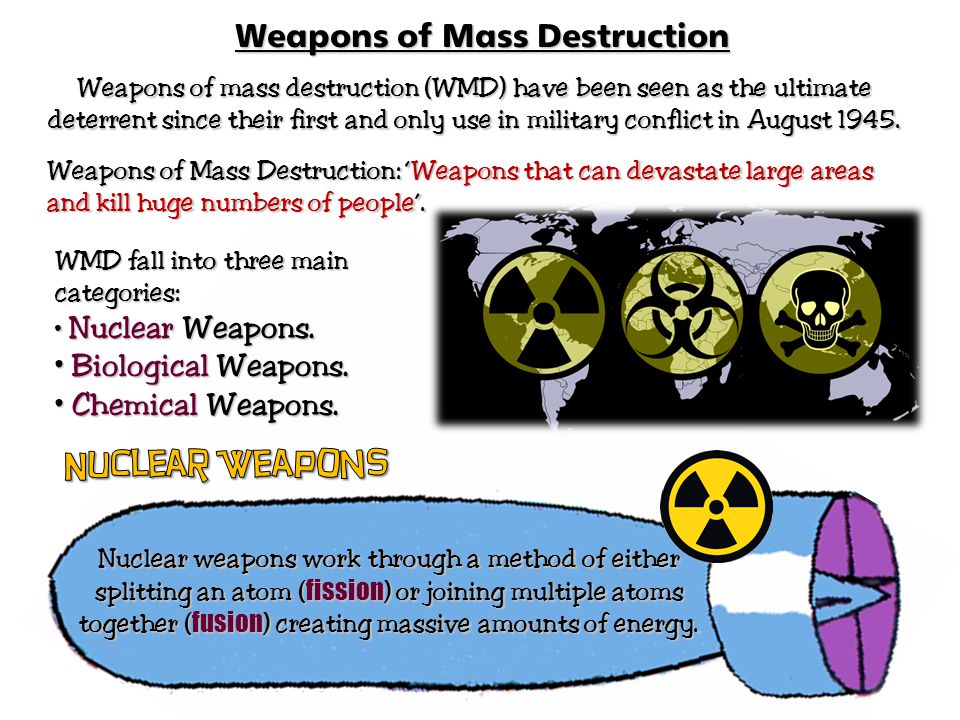The image features a poster titled "Weapons of Mass Destruction" in bold, underlined black lettering at the top. The text "Weapons of Mass Destruction (WMD) have been seen as the ultimate deterrent since their first and only use in military conflict in August of 1945" appears in a fun, kid-friendly font. Within the poster, the phrase "weapons that can devastate large areas and kill huge numbers of people" is highlighted in red. 

The poster organizes WMD into three main categories: nuclear weapons, biological weapons, and chemical weapons. The words "nuclear," "biological," and "chemical" are emphasized in a dark purple color, while "weapons" is in black. Further detailed text explains that nuclear weapons operate by either splitting an atom (fission) or joining multiple atoms together (fusion), processes that create massive amounts of energy. Within this section, the words "fission" and "fusion" are also highlighted in purple.

Visually, the poster includes a rectangular image on the right side featuring three icons centered on a globe or map of the world. These icons are circular and are all in green and black: a hazardous symbol, a biohazard symbol, and a skull and crossbones. Additionally, a yellow and black biohazard icon appears near the bottom of the poster.